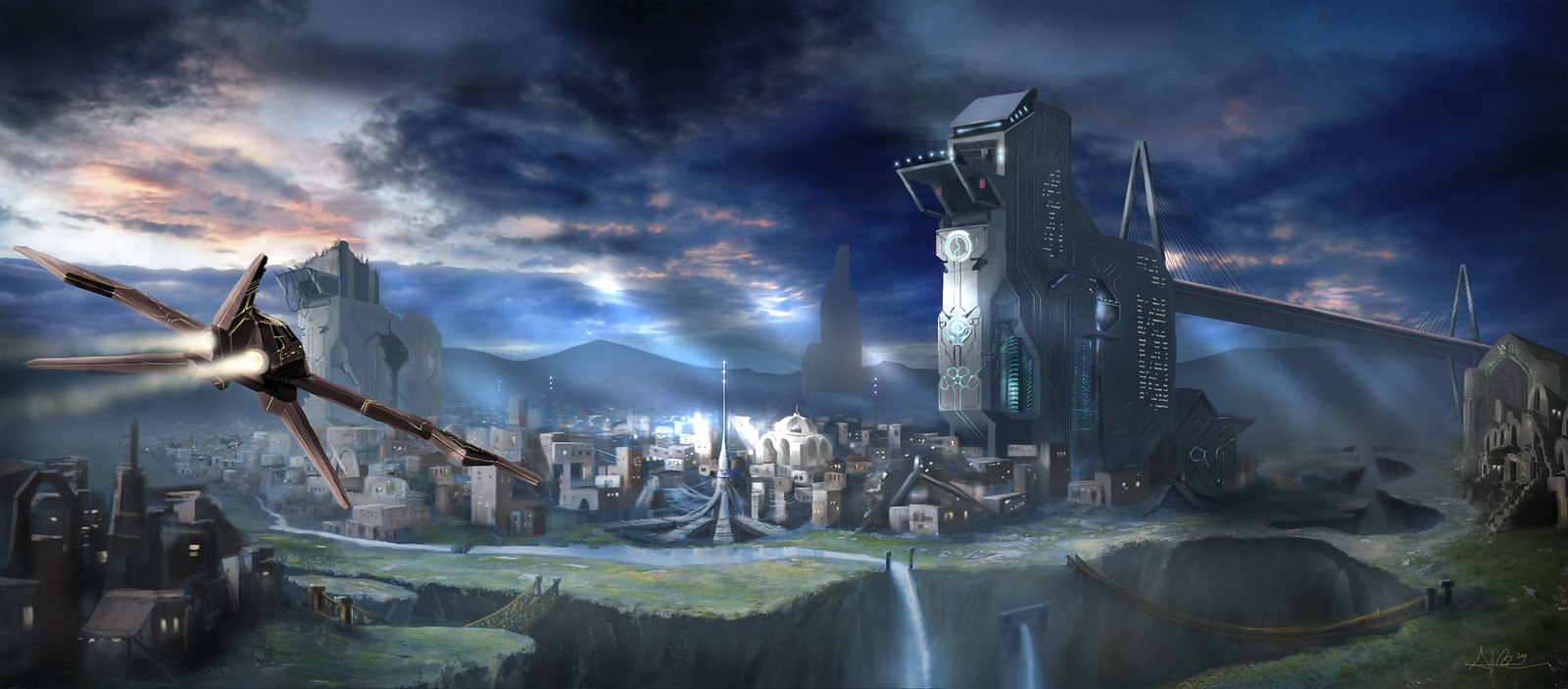The image depicts an artist's rendition of a futuristic town set within a valley surrounded by mountains under a multicolored sky. Prominent features include a mix of large gray futuristic buildings with interconnected metal platforms and smaller housing units, forming a cohesive community-like structure. In the forefront, a large crack in the ground channels a stream of water running off a cliff. A wooden swing bridge crosses this crack, leading to a grassy area. The left side of the image features a small spacecraft, underscoring the science fiction theme. The sky is a patchwork of cloudy blues, oranges, and purples with glimpses of pink and peach sunlight filtering through, providing a dramatic backdrop. Additionally, a unique structure resembling a lighthouse, possibly for bridge controls, stands out at the end of the bridge.